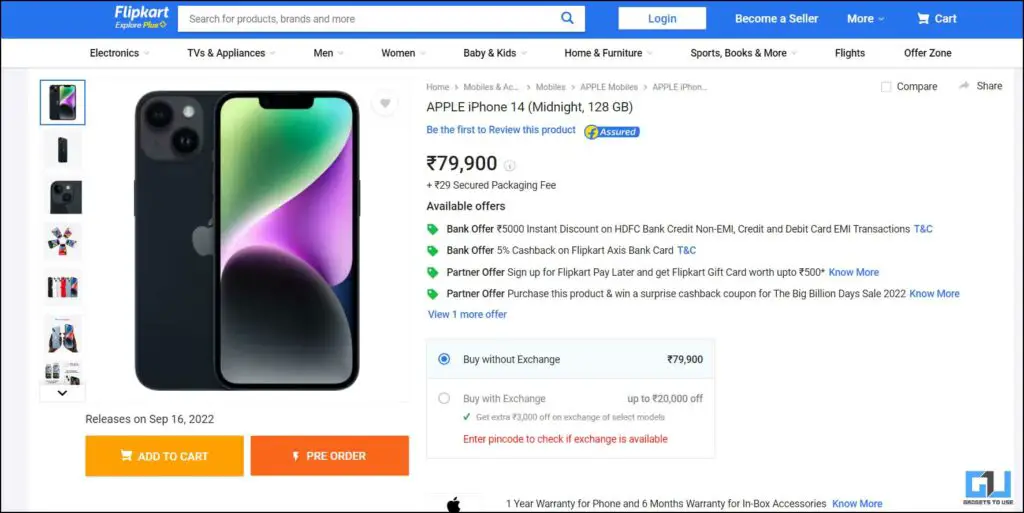**Detailed Caption:**

The webpage featured is for purchasing a phone on Flipkart, with a sleek blue-themed user interface. At the top, there's a blue navigation bar which includes a white search bar for searching products, brands, and more. Adjacent to the search bar, there's a white login button with blue text that reads "Login," followed by "Become a Seller," "More," and "Cart" all in white text set against the blue background.

Below this navigation bar, a secondary white horizontal menu bar provides categories including Electronics, TVs & Appliances, Men, Women, Baby & Kids, Home & Furniture, Sports Books & More, Flights, and Offer Zone. Each category, except for Flights and Offer Zone, has a pull-down context menu for further navigation.

The primary item displayed on the page is the Apple iPhone 14 in Midnight color with a storage capacity of 128 GB. The product listing shows it is Flipkart Assured, priced at ₹79,900. There are purchasing options available: "Buy Without Exchange" at ₹79,100 and "Buy With Exchange" offering up to ₹20,000 off. To the left of the product details, several images of the iPhone 14 are displayed. 

Beneath the product information, there is an orange "Add to Cart" button with white text, and next to it, an orange-colored "Pre-order" button with white text on a dark orange background. This detailed page layout guides users through the process of purchasing the latest Apple iPhone 14.